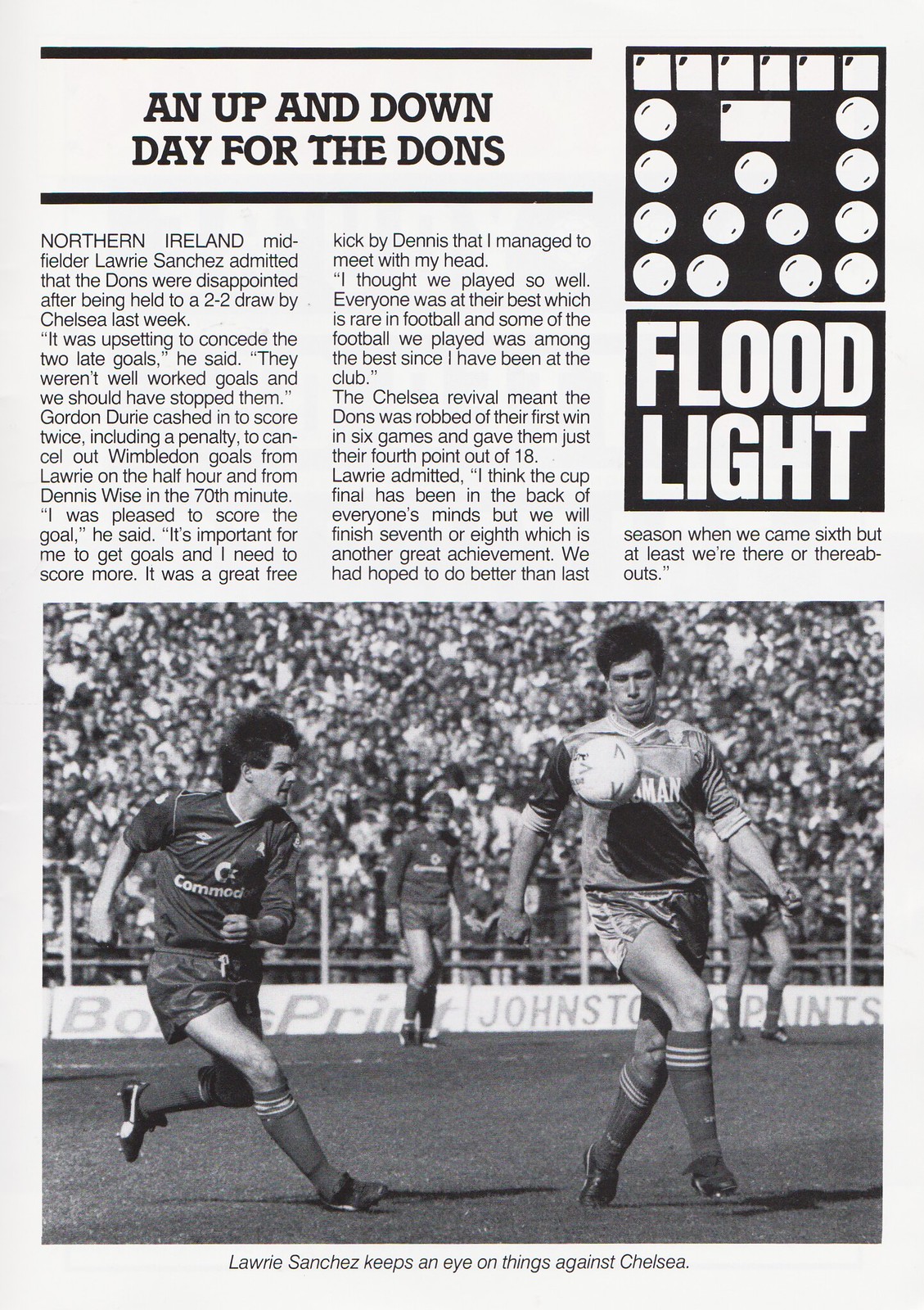This black-and-white scan of a page from a newspaper or team magazine features an article prominently titled "An Up and Down Day for the Dons." The publication, possibly named "Floodlight," is indicated by an emblem on the right side consisting of a stylized drawing of lights with the word "Floodlight" beneath it. The centerpiece is a large photograph of a soccer stadium filled with a cheering crowd. In the image, two men from opposing teams—one preparing to kick a soccer ball and the other running towards him—are captured in action, with their cleats and long socks clearly visible. The background shows two additional players and rows of spectators. The page is formatted with the text of the article in three columns, all detailing the match between Chelsea and the Dons, and beneath the image is a caption reading, "Lori Sanchez keeps an eye on things against Chelsea."